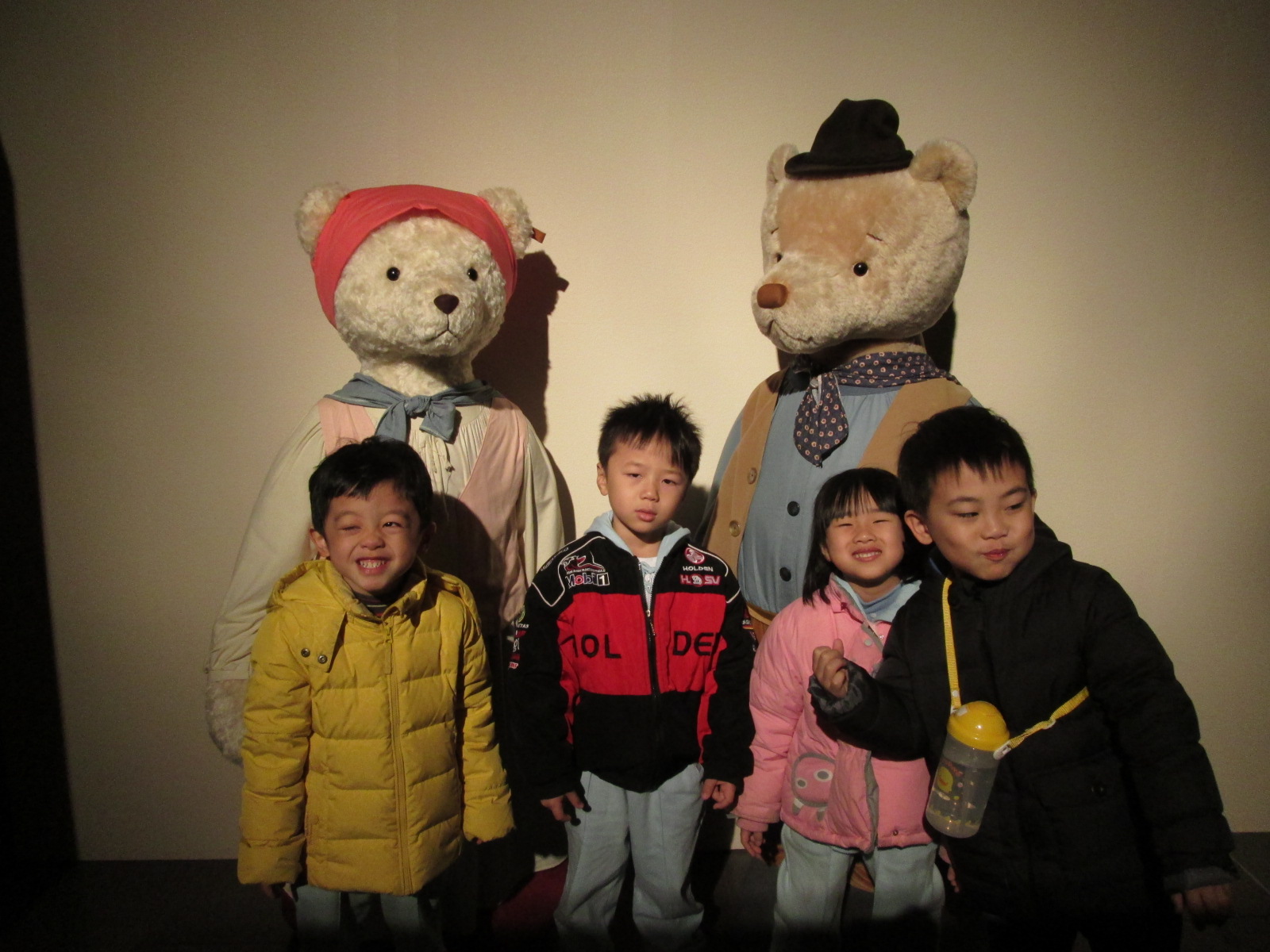This color photo captured indoors features four Asian children, lined up in front of two life-size stuffed bears, standing against a well-illuminated white wall. The two bears tower over the children, adorned in distinct and detailed costumes. The bear on the left is dressed in a red bandana, a blue neckerchief, a pink apron, and appears to be female, while the bear on the right sports a black hat, a purple neckerchief, a tan vest, and a blue shirt, depicting a male.

The children, all dressed in winter attire, show a range of expressions. The boy in the far left, wearing a yellow coat, is smiling with one eye winking. Next to him, a boy in a black and red coat and blue jeans looks unimpressed. The girl beside him, donning a pink coat and blue jeans, smiles with her eyes partially closed. Lastly, the boy on the far right, dressed in a black coat, stands with a cheerful demeanor, carrying a thermos with a yellow strap across his chest. Despite the bright flash illuminating the scene, which suggests an indoor, well-lit environment, the two children on the edges are looking off-camera, adding a candid touch to the otherwise posed photograph.